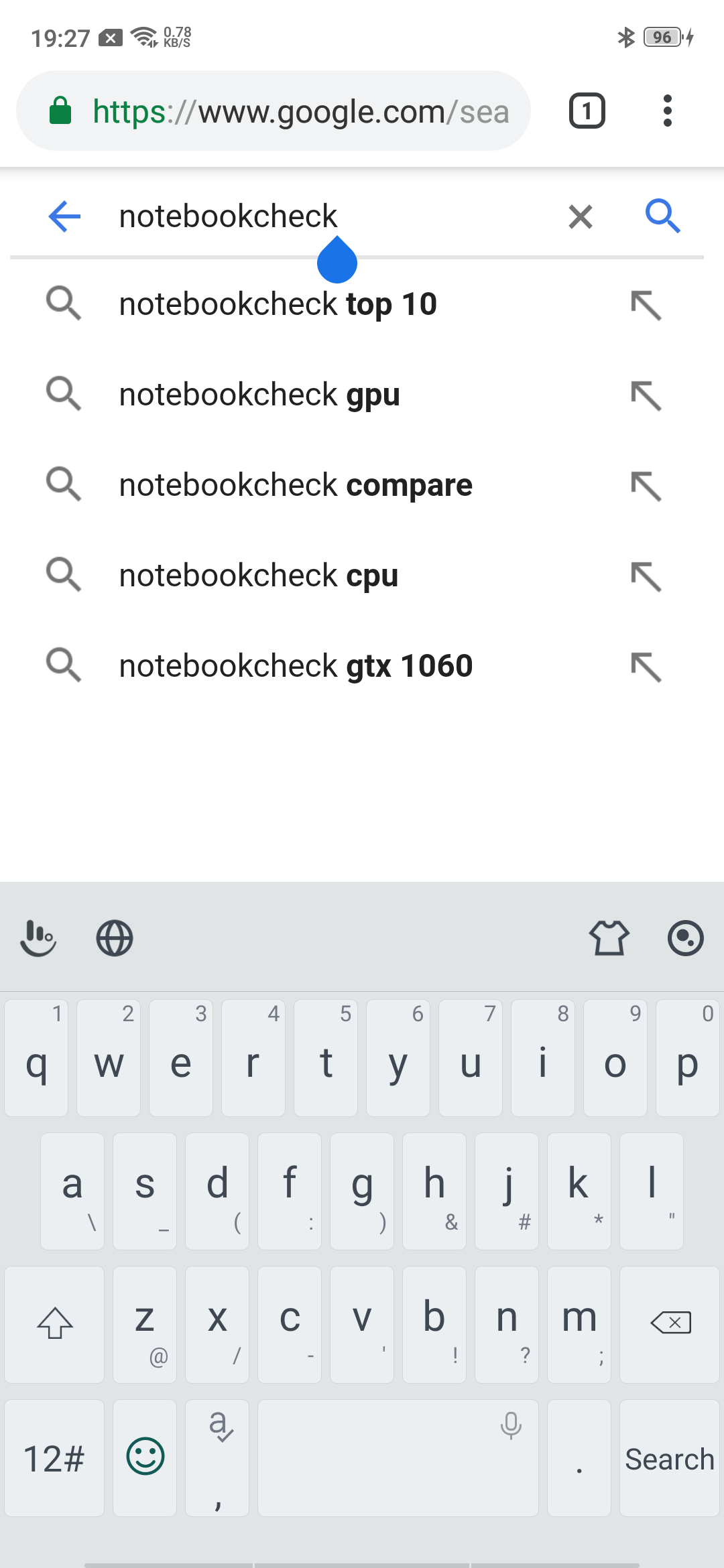A screenshot of the Google search homepage featuring the URL "https://www.google.com" at the top. The search bar displays the text "notebook check" with autocomplete suggestions listed below, including "notebook check top 10 notebook GPU," "notebook check compare notebook CPU," and "notebook check GTX 1060." The screen's lower portion shows the on-screen keyboard interface.